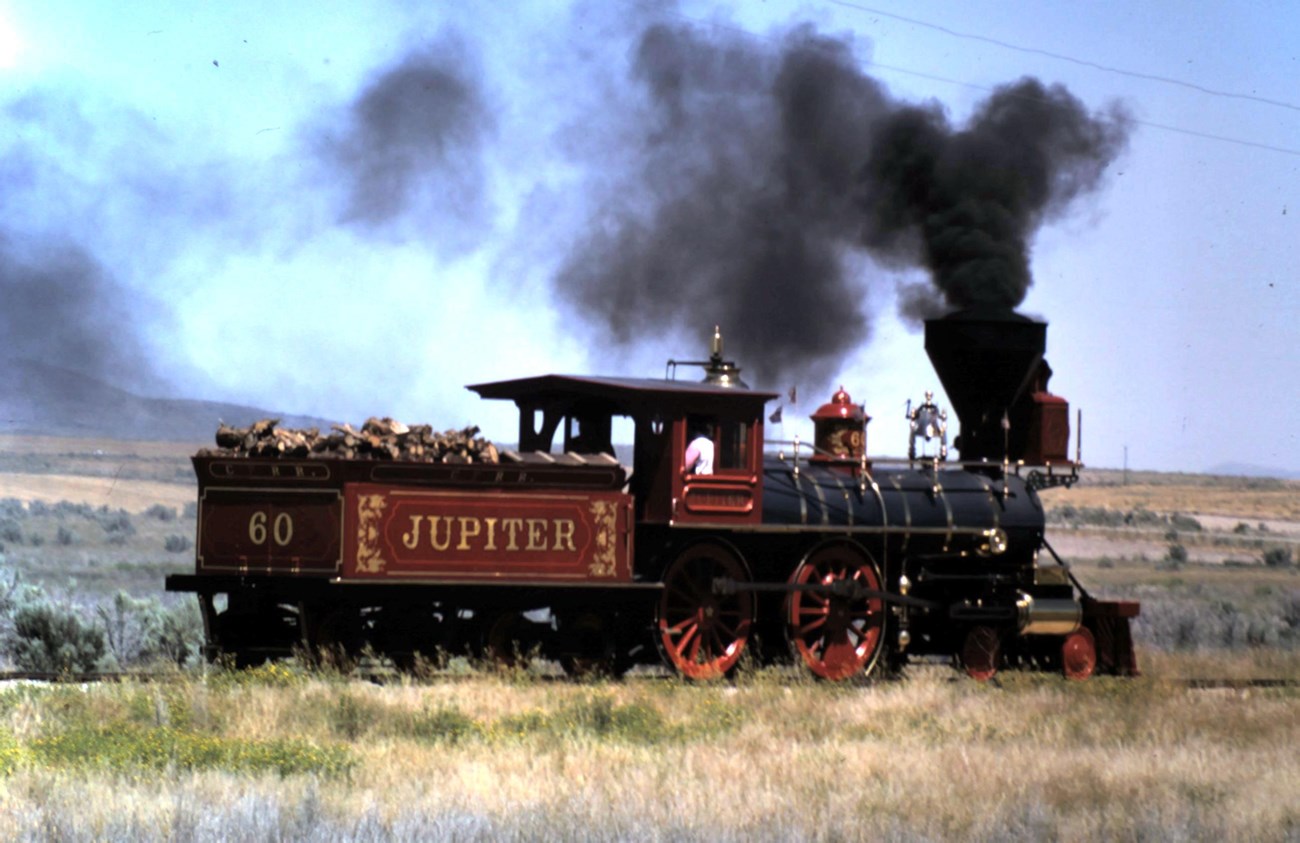In this outdoor image, the foreground showcases the front engine of an old, black steam train with a prominent black smokestack emitting thick, black smoke. The engineer's cab and the spokes of the large wheels are painted a dark red. Attached to the back of the engine is a small, open car filled with wood, bearing the name "Jupiter" in gold letters on its side and the number "60" in gold on its rear. Surrounding the train, the background reveals a vivid blue sky, intersected at the upper left by a power line, and a dark-colored mountain or hill on the left side. Below this terrain lies an expansive prairie adorned with light brown and green fields dotted with sagebrush, trees, and bushes. The prairie grass appears slightly blurred, lending a sense of depth to the landscape. The overall aesthetic evokes a vintage or historical feel, reminiscent of a scene from a Western movie or old TV show.